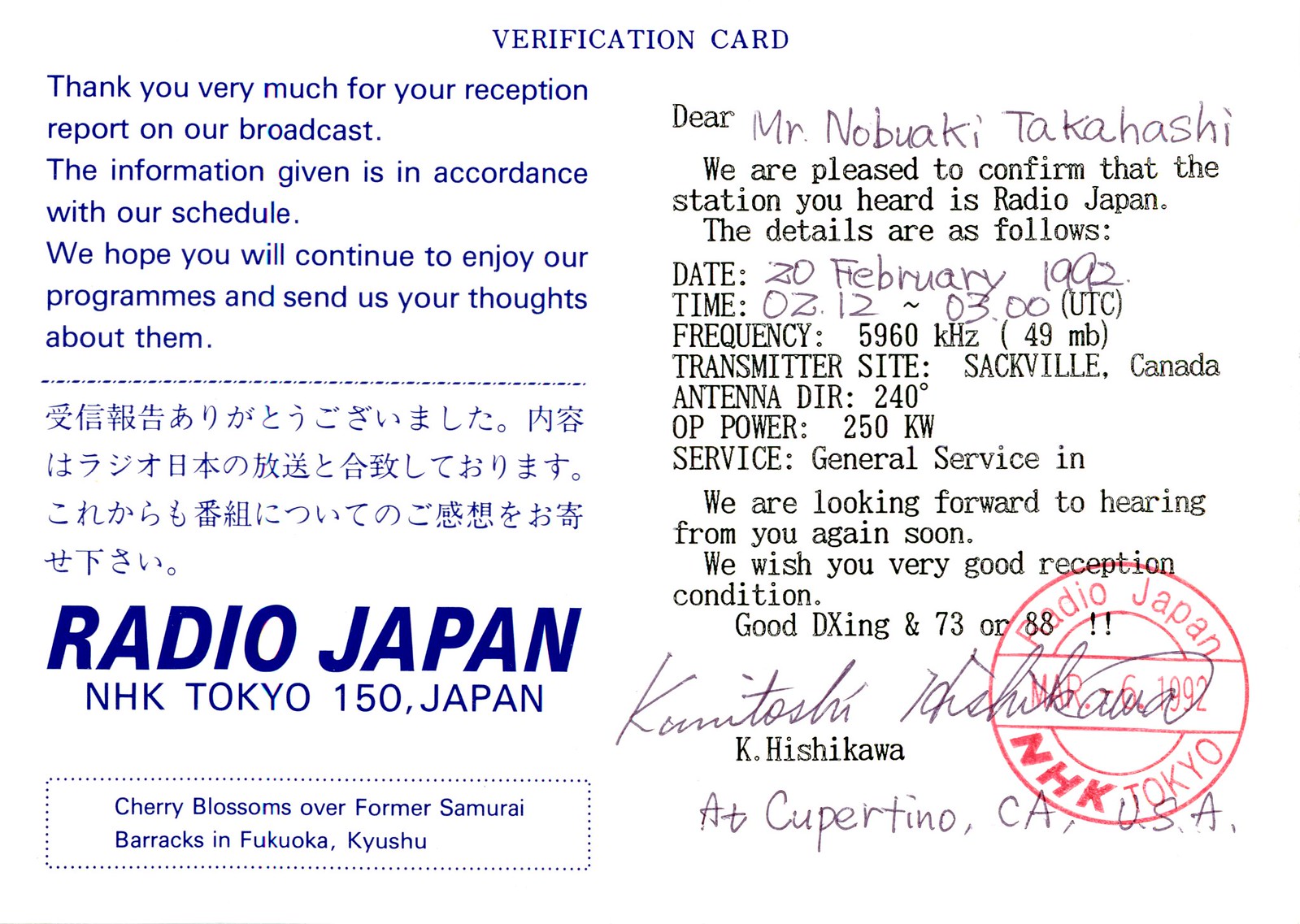The image depicts a detailed verification card with a white background. At the top, it says "Verification Card" and to the left, a thank you message is written in a slightly purple font: "Thank you very much for your reception report on our broadcast. The information given is in accordance with our schedule. We hope you will continue to enjoy our programs and send us your thoughts about them." Below this message, there is a dashed line followed by a paragraph in Japanese. Large bold blue letters spell out "Radio Japan," and underneath, it reads "NHK Tokyo 150, Japan."

To the right side of the card, it’s addressed to Mr. Nobuaki Takahashi with a typed message confirming the reception report: "We are pleased to confirm that the station you heard is Radio Japan. The details are as follows: Date: 20th February 1992; Time: 0212 - 0300 UTC; Frequency: 5960 kHz (49 MB); Transmitter Site: Sackville, Canada; Antenna Direction: 240°; Power: 250 kW; Service: General Service. We look forward to hearing from you again soon. We wish you good reception conditions, good DXing, and 73." The card is signed by K. Hishikawa and features a postmark indicating it was sent from Radio Japan NHK Tokyo on March 6, 1992. At the bottom within a dashed rectangle, it mentions "Cherry blossoms over former samurai barracks in Fukuoka, Kyushu."